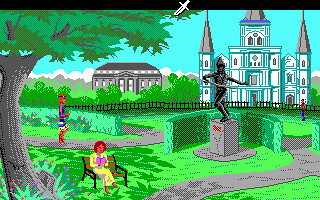This heavily pixelated, computer-generated image—likely a still from a video game or digital rendering—depicts a lively park scene. Central to the image is a statue with a person atop, brandishing a sword, surrounded by meticulously groomed bushes. A woman in a yellow dress sits on a bench beneath a large green leafy tree, engrossed in reading a book. Nearby, a jogger in shorts and a blue shirt is seen on a meandering grey walkway that circles the statue and flowers. In the background on the right, a majestic white castle with three turrets—two with gray roofs and the center one with a purple-trimmed roof—dominates the skyline. To the left of the castle in the far distance, there is a dark grey structure that might be a mausoleum or a government building. The scene is set against a bright blue sky, adding to the vibrant atmosphere of the park.